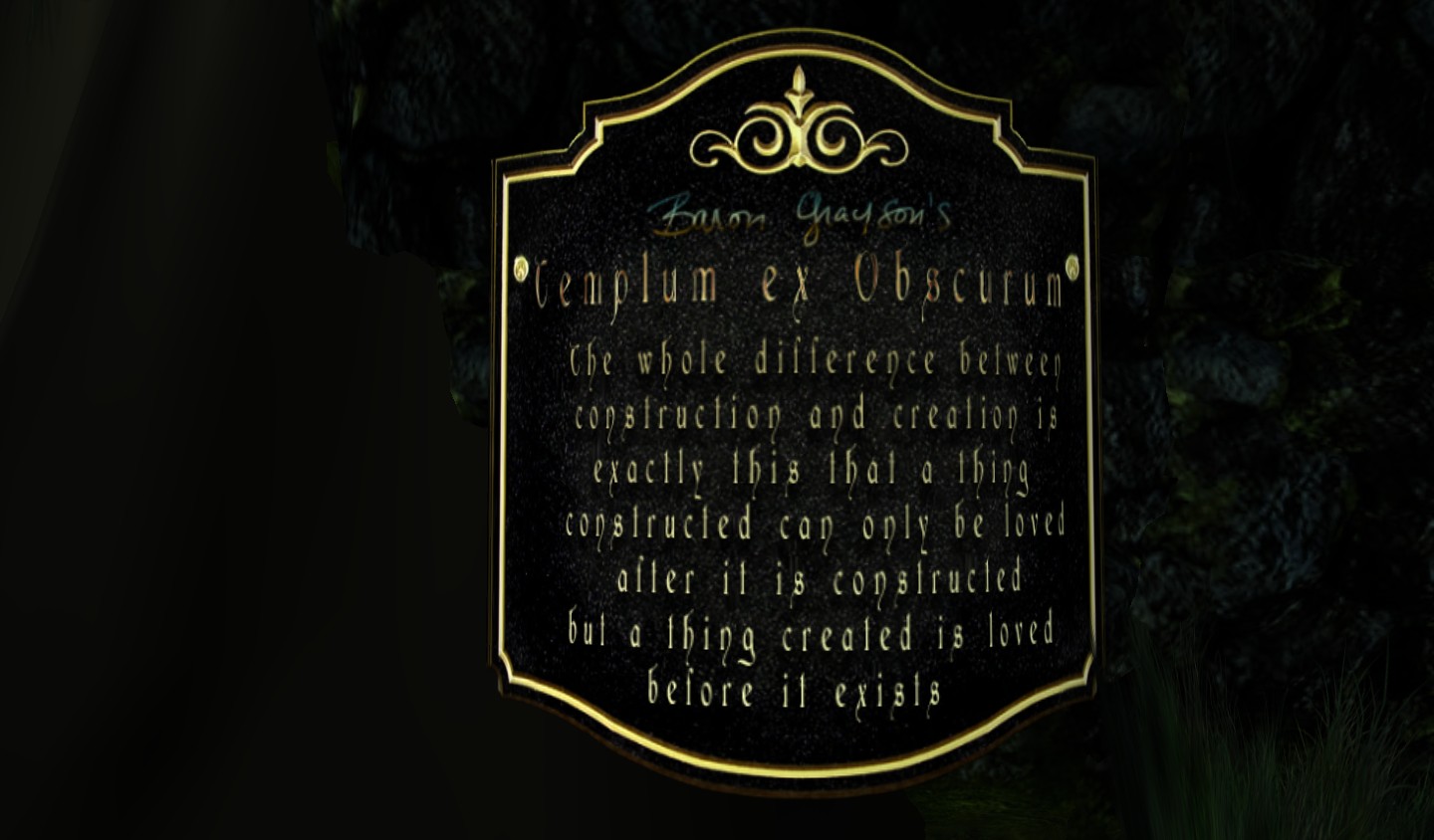The image depicts an elegantly designed plaque set against an all-black background. The plaque has a rounded design bordered with gold trim, featuring an insignia or emblem at the top, adding to its posh and high-class appearance. Surrounding the plaque are green leaves, suggesting a natural or artistic environment. The plaque displays a thoughtful quote in gold cursive that reads, "Templum Ex Obscurum, the whole difference between construction and creation is exactly this: that a thing constructed can only be loved after it is constructed, but a thing created is loved before it exists." The top of the plaque inscribes “Grayson's,” hinting that it may be attributed to or created by someone named Grayson. The overall aura of the image is one of sophistication and contemplation.